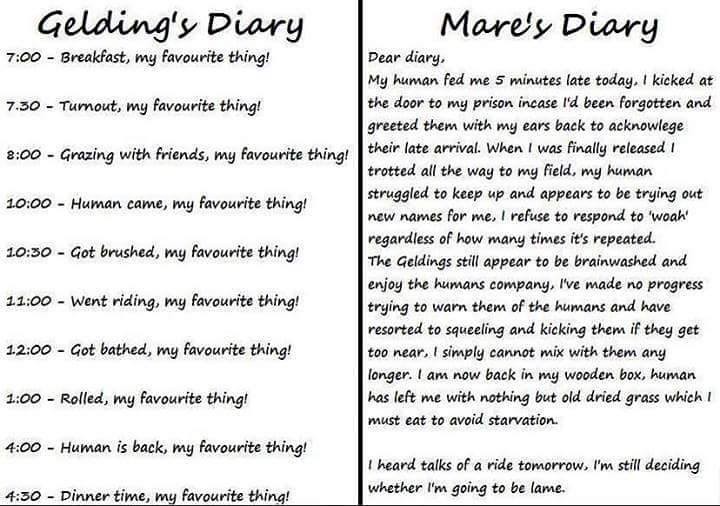The image features two adjacent diary pages against a pure white background, both presented in an elegant black font. The left page is titled "Gelding's Diary" and outlines a meticulously scheduled day. It begins at 7:00 AM with "Breakfast, my favorite thing," followed by "Turnout, my favorite thing" at 7:30 AM, then "Grazing with friends, my favorite thing" at 8:00 AM, continuing with "Human came, my favorite thing" at 10:00 AM, "Got brushed, my favorite thing" at 10:30 AM, "Went riding, my favorite thing" at 11:00 AM, "Got bathed, my favorite thing" at 12:00 PM, and culminating in "Dinner time, my favorite thing" at 4:30 PM.

The right page is labeled "Mare's Diary" and opens with "Dear Diary." It describes a pet's disgruntlement over being fed five minutes late, prompting it to kick at the door of its enclosure and greet its human with ears pinned back in displeasure. It mentions a brisk trot to its field, causing its human to struggle to keep up and refusing to respond to a new name being tried out by the human. The entry concludes with the pet overhearing plans for a ride the next day and musing over whether to pretend to be lame to avoid it.